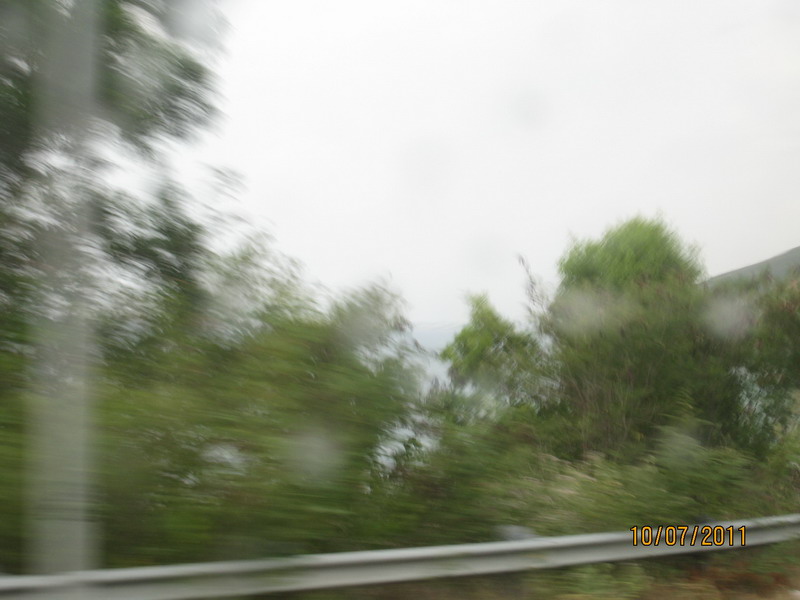This rectangular image, only slightly wider than it is tall, captures a blurry roadside scene. Spanning from the lower left corner to a point slightly above the bottom right corner, the image features a single, metal gray highway guardrail, angled upwards at approximately 15 to 20 degrees. In the lower right corner, the guardrail overlaps with an orange timestamp marking "10 07/2011," possibly indicating October 7, 2011, or July 10, 2011, depending on regional date formats.

The greenery around the guardrail is lush and varied. On the lower right corner, beneath the guardrail, and extending above it, we see medium green foliage. The left side of the image is dominated by trees reaching all the way to the top, with darker green shades prevalent. On the right side, the greenery reaches only about halfway up the image, revealing the skyline.

Partially obscured by the foliage on the right side, a whitish structure is visible, suggesting either a building or a billboard with some indiscernible text. Above, the sky appears almost entirely white with a light gray tint, contributing to the overall blurriness of the scene.